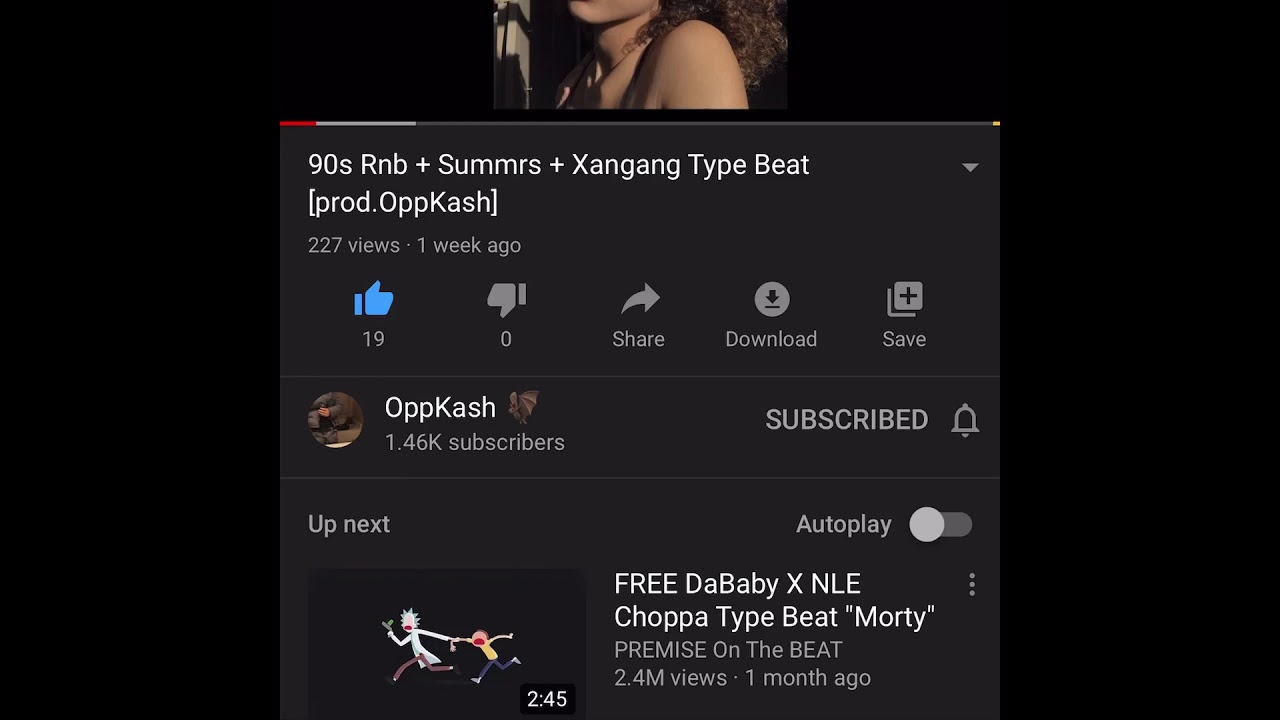The image features a solid black background with a prominent central element. At the upper center, there's a partial depiction of a woman’s shoulder and chin; she's wearing a tank top and has dark, curly hair that cascades down to her shoulders. Her face is not visible.

Dominating the center of the image is a large pop-up box, also set against a black backdrop. The top section of this box contains a bar partially colored in red and gray. Below the bar, white text reads: "90s R&B + SUMMRS + XANGANG type beat (Prod. OPP Cash)." Further details indicate the video has garnered "227 views one week ago" with "19 thumbs up" and "0 thumbs down." Below this information are buttons labeled "Share," "Download," and "Save."

The channel name, "Opcash 🦇," is displayed, showing that the channel has 1.46k subscribers and that the viewer is subscribed. 

Below the main pop-up box, the image indicates an "Up next" section featuring a thumbnail with another black background. This thumbnail shows characters Rick and Morty running, promoting a video titled "Frida Baby - NLE Choppa Type Beat 'Morty' (Prod. Premise on the Beat)" which has "2.4 million views one month ago."